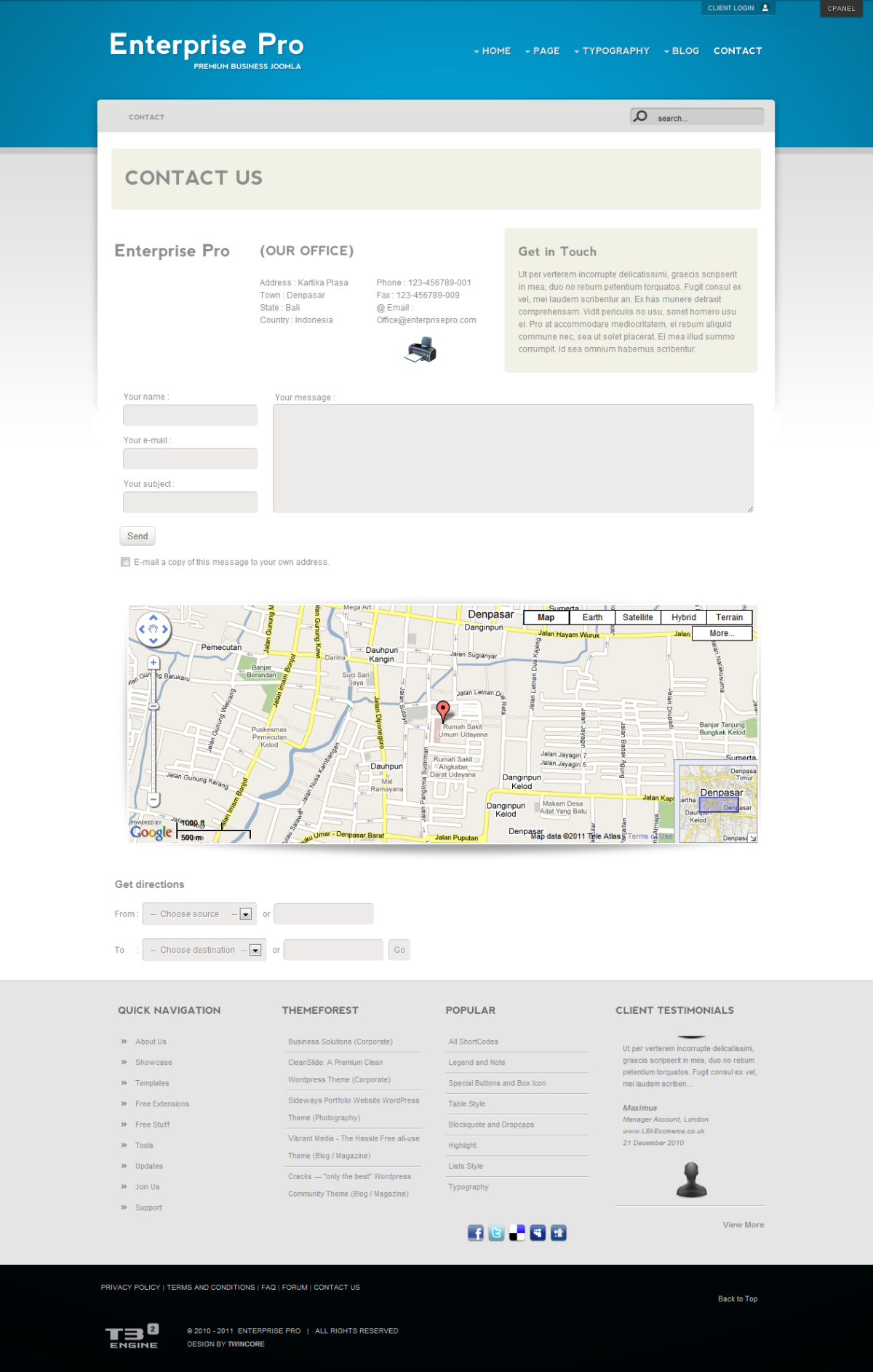This image is a screenshot from the "Contact Us" page of the Enterprise Pro website. At the top left of the page, the heading "Contact Us" is prominently displayed, indicating this section’s purpose. The main content area of the page includes a bar labeled "Enterprise Pro," beneath which the office address and phone number are listed. Below this information, there are interactive fields where users can input their name, email address, subject, and message. A "Send" button is positioned near these fields, with a checkbox located directly underneath it. At the bottom of the page, a map is displayed, pinpointing the location of the Enterprise Pro office. This layout provides users with all necessary contact details and a convenient way to reach out.